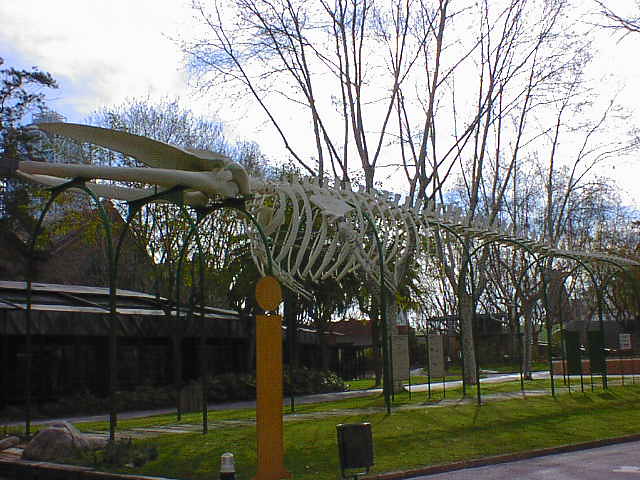The photograph captures an outdoor exhibit on a gray, fall day, featuring the skeleton of a prehistoric creature, likely a plesiosaurus, displayed prominently on black metal arches that elevate it above the ground. The plesiosaurus bones, white and striking, span the middle of the image, creating an awning-like effect over the grassy area beneath. The long tail and elongated skull with a massive mouth are particularly notable, suggesting a sense of grandeur and awe. There is a sidewalk that curves from the lower left to the right, passing underneath the skeletal display, which allows visitors to walk directly beneath the arches.

In the middle foreground, a yellow pole stands at the corner where the grassy area meets a curb, while another brown post attached to one of the arches possibly offers information about the exhibit, though the text is not legible. Trees with bare branches, indicating the fall season, frame the scene, and a row of buildings, possibly one-story structures, forms the background. These buildings are positioned on the left and right sides, contrasting with some non-descript structures on the right. The trees in the middle right of the photo stretch up to the top, adding vertical elements. 

Additionally, there are green poles within the grassy area, and what appears to be ornate fence-top designs run horizontally through the image toward the right, ending in three white protrusions with curling details beneath them. A wastebasket can be seen towards the bottom center of the picture, contributing to the park-like ambiance of this setting, which might be within or adjacent to a museum.